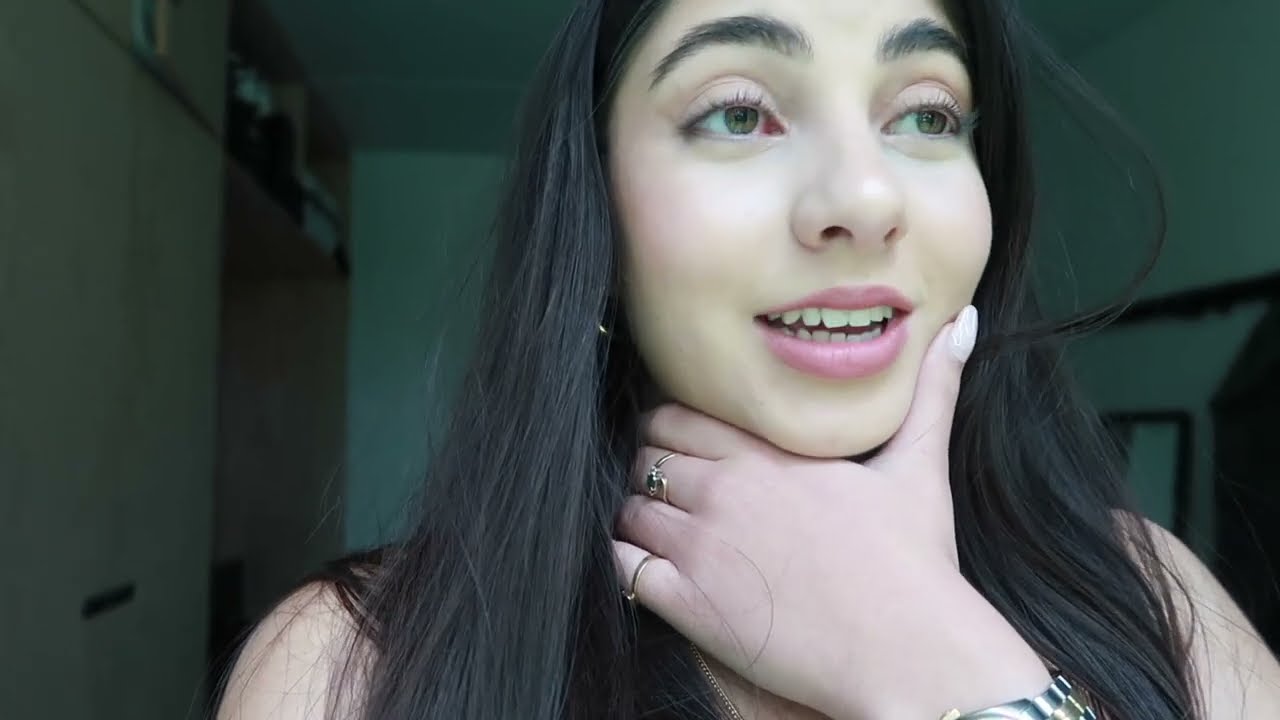The photograph, taken indoors, captures a beautiful woman in her mid-20s, with fair skin, long, black hair that falls past her shoulders, and thick black eyebrows accentuating her hazel eyes. She wears light pink eyeshadow and black mascara, with pink lipstick highlighting her slightly open mouth, displaying both her upper and lower rows of teeth in what appears to be a mid-sentence expression. 

The woman is gazing to the side, possibly towards a computer or the distance, with her left hand gracefully positioned under her chin, her thumb resting against her cheek, and her fingers curling around her neck. On her left wrist, partially obscured by the frame, is a silver stainless steel watch with a gold band running through the middle. She also sports a long white manicure on her thumb, and wears two rings: a thin gold ring on her middle finger and another ring on her pinky.

The background appears somewhat blurry, suggesting the photo was taken at close range, possibly with a webcam. The walls behind her are a mix of white and blue, with a stained yellow and white section to the left and a slightly open door behind her. To the right of her left shoulder, there is a mirror, hinting that she might be in her bedroom.